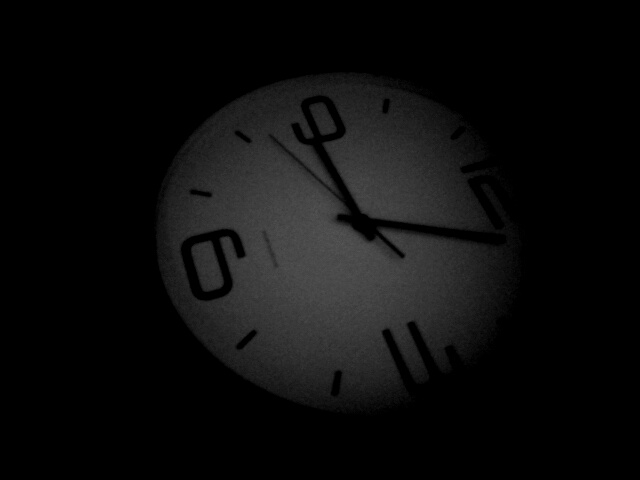The photograph captures a circular wall clock against a completely black background, suggesting a very dark room potentially illuminated by a camera flash. The clock, featured in the center of the image, has a white face with black numerals and hands, including the minute and second hands. The clock displays the time as 9:02, though it is slightly tilted to the right, causing the 12 to appear on the right side and the 6 on the left. Only the numerals 12, 3, 6, and 9 are marked on the clock face, while the other hours are indicated by small black lines. The clock's brand name is also present but not legible due to the small font size. The image appears blurred, likely due to low light conditions during the photo's capture.